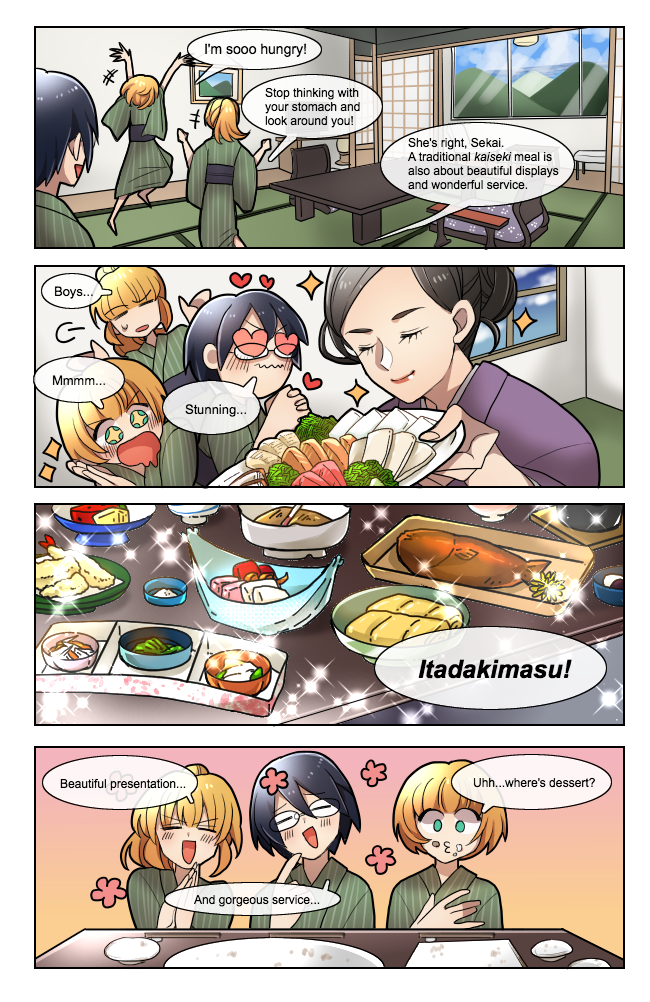This comic strip features a traditional kaiseki meal across four illustrated panels. In the first panel, three women are depicted from the back, dressed in green kimonos with black sashes, in a room with an Asian-style low table and a view of hills and clouds outside. They express their anticipation and appreciation for the meal: "I'm so hungry," says one. "Stop thinking with your stomach and look around you," replies another. The third adds, "She's right, Siki. A traditional kaiseki meal is also about beautiful displays and wonderful service."

The second panel shows four characters admiring the beautifully presented food. A woman in the foreground, with dark hair pulled back, holds a plate laden with various foods. The three visible figures to the left have exaggerated expressions of delight, with one saying, "Boys," another, "Mmm," and the third, "Stunning," while hearts and stars float around their heads.

In the third panel, a detailed shot of the table reveals an array of Asian cuisine, including fish, bread, tofu, and soup, along with the exclamation "Itadakimasu!"

The final panel captures the three women now facing forward, surrounded by flowers and looking thrilled. They praise the meal: "Beautiful presentation and gorgeous service," one says, followed by another inquiring, "Oh, where's dessert?"